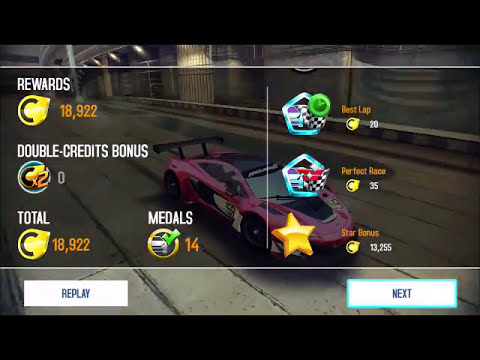This image is a screenshot from a video game featuring a race car. The scene is bordered by black trims at the top and bottom, framing the main picture. The focus is a race car, angled slightly to the right, with a distinctive black fan tail at the back. The car is in a dark reddish-pink or purplish hue, with dark windows, a black top, and some black markings on the front hood. On the passenger side, there's a prominent white area displaying the black number "59."

In the upper left section of the screen, the word "REWARDS" is displayed in white, capital letters. Below this, a yellow icon with a black "C" and the number "18,922" in orange. The phrase "double credits bonus" appears in white lettering underneath. Next, a circular icon labeled "C times two" shows a value of zero. Further down, the word "total" is followed by the same yellow symbol with the black "C" and the number "18,922" in orange. To the right, the section marked "medals" contains a circular icon featuring a race car with a green check mark over it, along with the number "14."

On the right side of the screen, there are multiple highlights. First, a five-sided figure with a black and white checkered flag and a green circle, resembling a clock, is labeled "best lap" next to a smaller version of the yellow "C" icon with the number "20." Below, another five-sided figure with a turquoise outline features a checkered flag with a car, labeled "perfect race," followed by the yellow "C" icon and the number "35." Lastly, a section marked "star bonus" includes the yellow "C" icon and the number "13,255."

At the bottom of the image, two white, rectangular boxes are displayed. The one on the left, in blue capital letters, reads "replay," and the one on the right, outlined in a lime blue color, reads "NEXT" in black capital letters.